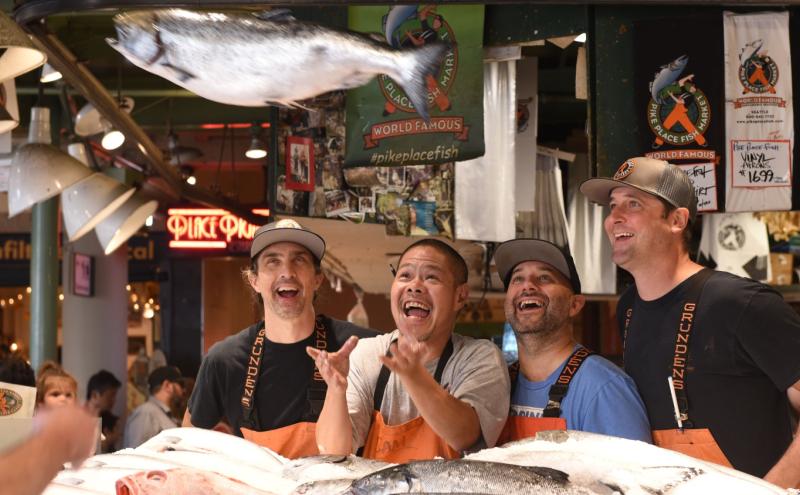In an indoor fish market bustling with activity and adorned with an array of colorful hanging banners and LED signage, four men are the main focus as they engage in the lively tradition of fish tossing. The men are positioned behind a table laden with a variety of fish on ice, all dressed in distinctive orange aprons emblazoned with the brand name "Grundens." Three of the men wear baseball-style hats, while the hatless one, positioned second from the left, appears to have just thrown a large, silver fish. His raised hands trace the motion of the fish as it sails through the air. The tallest of the group, standing a head above the others, is on the far right. Customers or additional market workers can be seen in the back left of the image, adding to the dynamic atmosphere, amidst a backdrop highlighted by bright lights and an assortment of banners and posters.